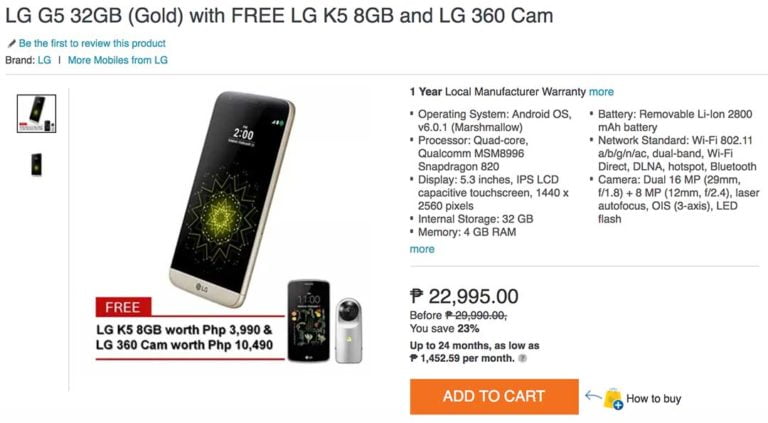Screenshot of an e-commerce website offering an LG smartphone package. At the top, there's bold text advertising an "LG G5, 32GB Gold" bundled with a "free LG K5, 8GB" and an "LG 360 Cam". The product image is displayed on the left side of the screen with a scrollable thumbnail menu beneath it for viewing additional images. To the right of the images, detailed product information is listed. The listing highlights that the LG G5 features a 5.3-inch display, runs on an Android system, is powered by a quad-core processor, includes 32GB of storage and 4GB of RAM, and comes with a one-year local manufacturer warranty. Additional sections provide more data about the battery, network, and camera capabilities. The item is priced at $22,995 in a foreign currency, and there is an "Add to Cart" button prominently displayed. The site layout and shopping features resemble those of major platforms like Amazon or eBay, though it is hosted by a different online marketplace.